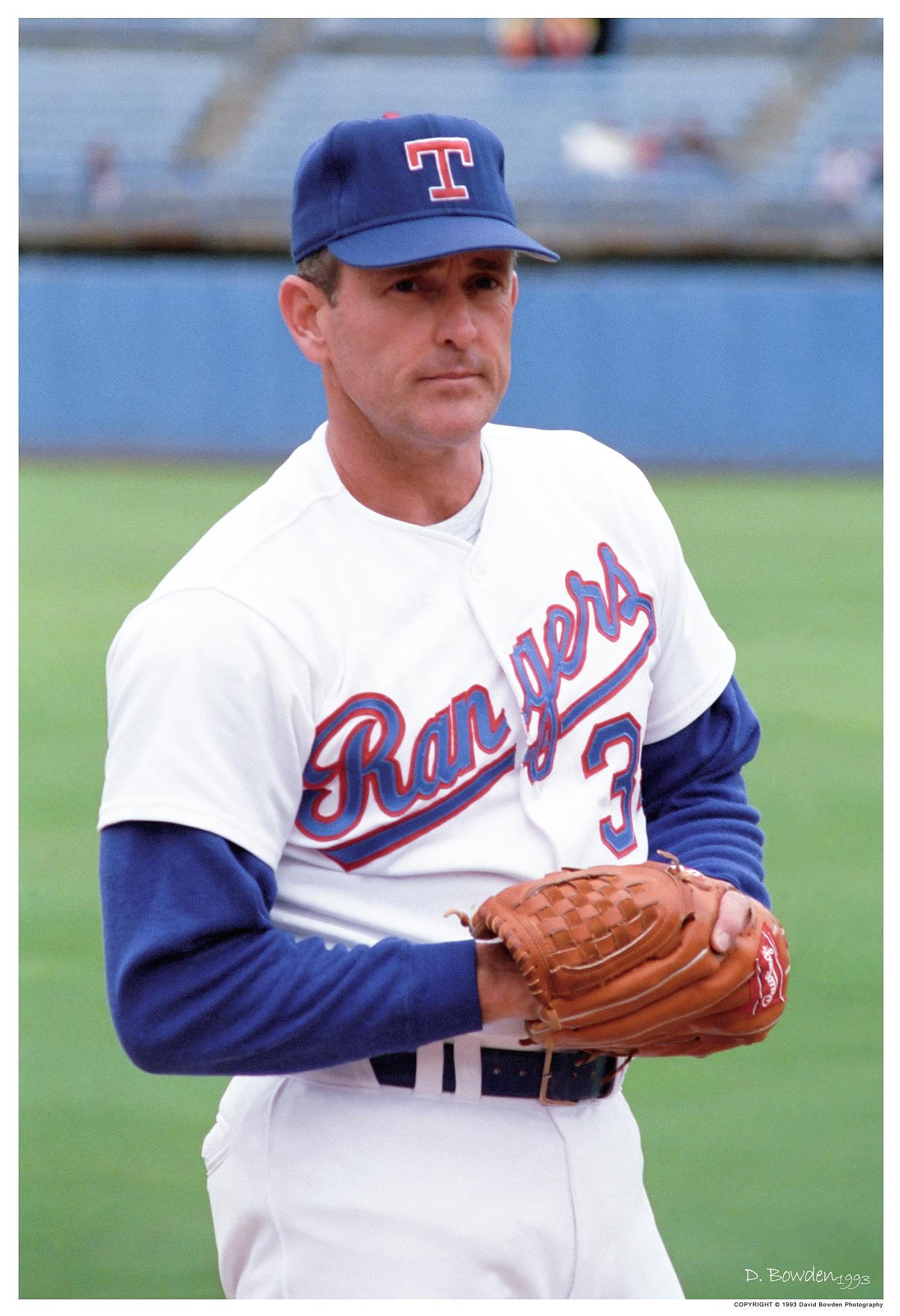In this photograph, we see a baseball player standing outdoors on a baseball field, likely captured in the middle of the day. The player is centrally positioned in the image, clad in a white jersey with "RANGERS" written diagonally across his chest in blue font. He wears a blue cap emblazoned with a red 'T' and has blue sleeves under his uniform. The number "3" is visible on his left side. His right hand, enclosed in a tan Rawlings glove, is held near his chest as if grasping something, while his left hand also seems to be interacting with the glove.

Behind him lies a large, flat, grassy field, giving way to a blue outfield wall and blurry bleachers above it. The stands are sparsely populated, with indistinct blobs of color suggesting a few people present. The image also captures gray walkways and stairs between the bleachers. Some small, unreadable text, likely a signature and copyright information, appears on the image. The overall color palette includes shades of green, blue, white, red, brown, and black.